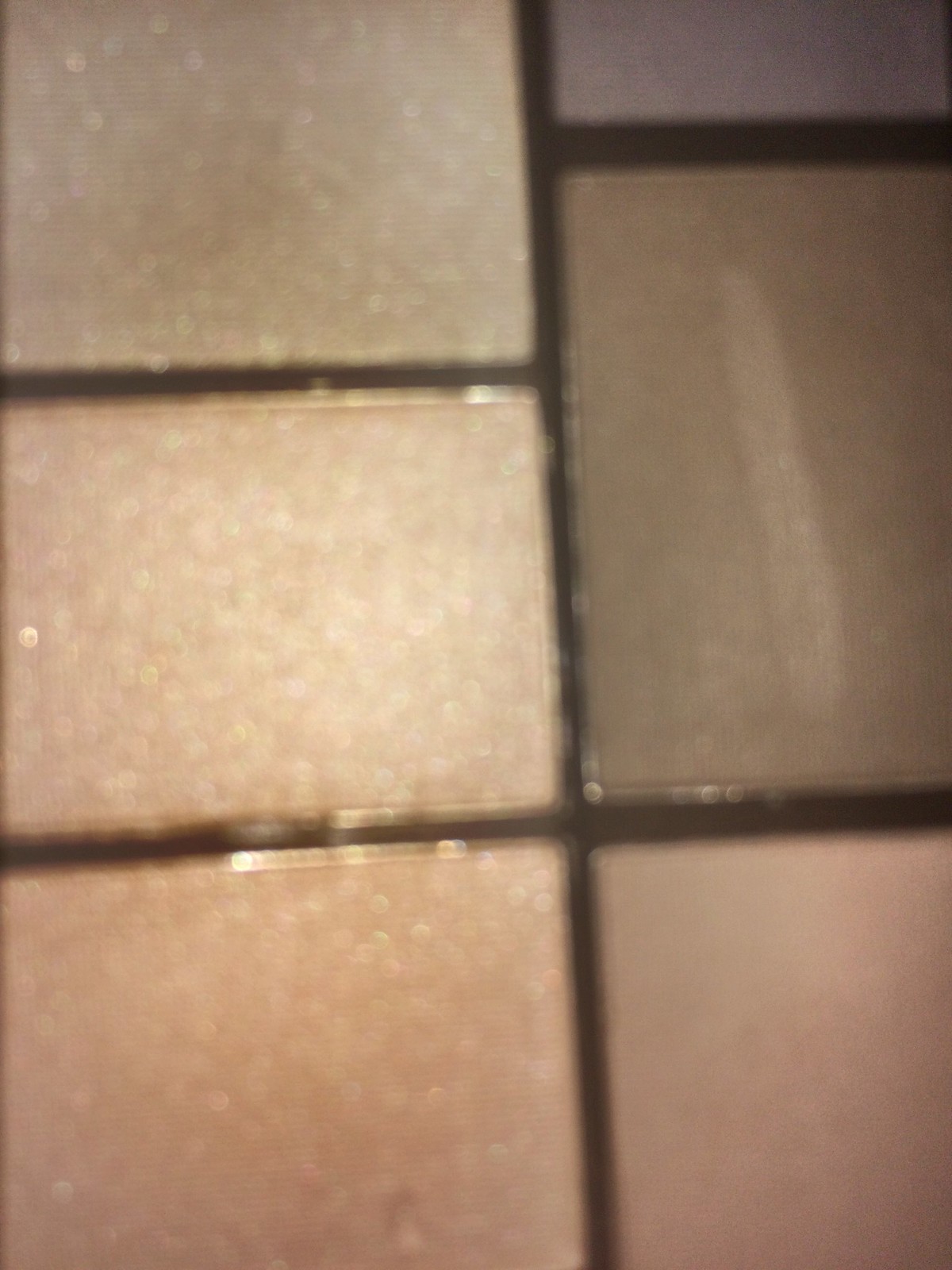This close-up, blurry photograph captures a section of a highly polished tile surface, possibly a wall or floor. The image focuses on an arrangement of six tiles in varying shapes and sizes, both square and rectangular. The tiles display a range of colors and textures, with a predominant palette of browns, including reddish-brown, gold-tinted brown, grayish-brown, and light tan with hints of pink. Notably, the upper left tile transitions from reddish on the left side to gold and then tan with a pinkish hue, while the upper right shows a blend of purple, brown, and pink, with a notable lighter brown smudge. The grout lines between the tiles are a consistent black or chocolate brown, adding contrast and framing to the scene. Despite the overall blurriness, the sheen on the tiles is noticeable, and the intricate color variations lend a rich, textured feel to the image.